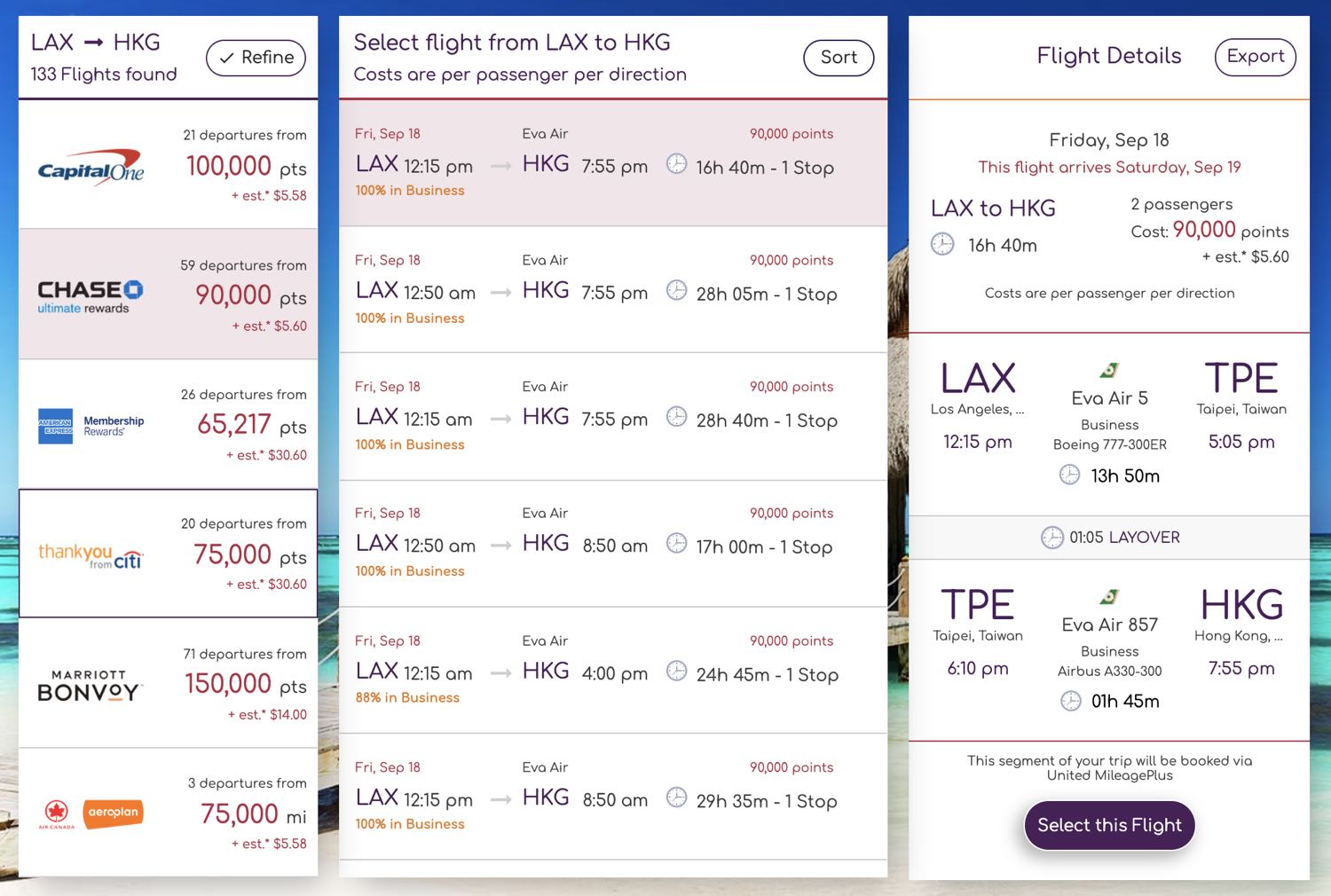**Detailed Caption:**

The image is a screenshot from a flight booking website, displaying listings for various flights. The webpage is divided into three main sections:

1. **Left Section: Flight Listings Overview**
   - At the top, there's a route indicator showing "LAX" with an arrow pointing towards "HKG," indicating a flight from Los Angeles (LAX) to Hong Kong (HKG).
   - Below this, a button labeled "Refine" with a checkmark suggests the user has applied filters.
   - The text "133 flights found" is displayed beneath the route information.
   - This section also showcases various credit card and loyalty program logos with corresponding point values:
     - Capital One: 100,000 points
     - Chase: 90,000 points
     - American Express: 65,217 points
     - Citi: 75,000 points
     - Marriott Bonvoy: 150,000 points
     - Aeroplan: 75,000 MI (miles)

2. **Center Section: Flight Selection**
   - This section is headed by the prompt "Select a flight from LAX to HKG" and a "Sort" button.
   - It notes that costs are per passenger per direction.
   - Several flight options are listed with identical dates "Fri, Sep 18," and varying departure and arrival times for LAX to HKG flights.
   - Each listing details include the departure time from LAX, the arrival time at HKG, the number of stops, and the total duration. There appear to be six selectable flights listed.

3. **Right Section: Flight Details**
   - The top displays "Flight details" with an "Export" button.
   - It provides specific information for a selected flight taking off on "Friday, Sep 18" and arriving on "Saturday, Sep 19."
   - Details include:
     - Route: LAX to HKG
     - Number of passengers: 2
     - Total flight duration: 16 hours and 40 minutes
     - Cost: 90,000 points plus $5.60 per passenger per direction

   - The itinerary is broken down:
     - Departure from LAX at 2:15 p.m. on EVA Air Flight 5 to TPE (Taipei, Taiwan), arriving at 5:05 p.m. on a Boeing 777-300ER (Business Class) with a duration of 13 hours and 50 minutes and a layover of 1 hour and 45 minutes.
     - Continuation on EVA Air Flight 857 from TPE to HKG, departing at 7:55 p.m. on an Airbus A330-300 (Business Class), with a flight duration of 1 hour and 45 minutes.
     - A note mentions that this segment of the trip will be booked via United MileagePlus.

   - At the bottom right, there is a dark purple, rectangular button with half-circle ends, labeled "Select This Flight."

**Background:**
   - A tropical destination background can be glimpsed behind the overlay of the three sections, showing a light blue or greenish-blue sea and a blue sky.

This detailed view provides comprehensive information about booking a flight from Los Angeles to Hong Kong, complete with credit card points, flight times, and detailed segment information.